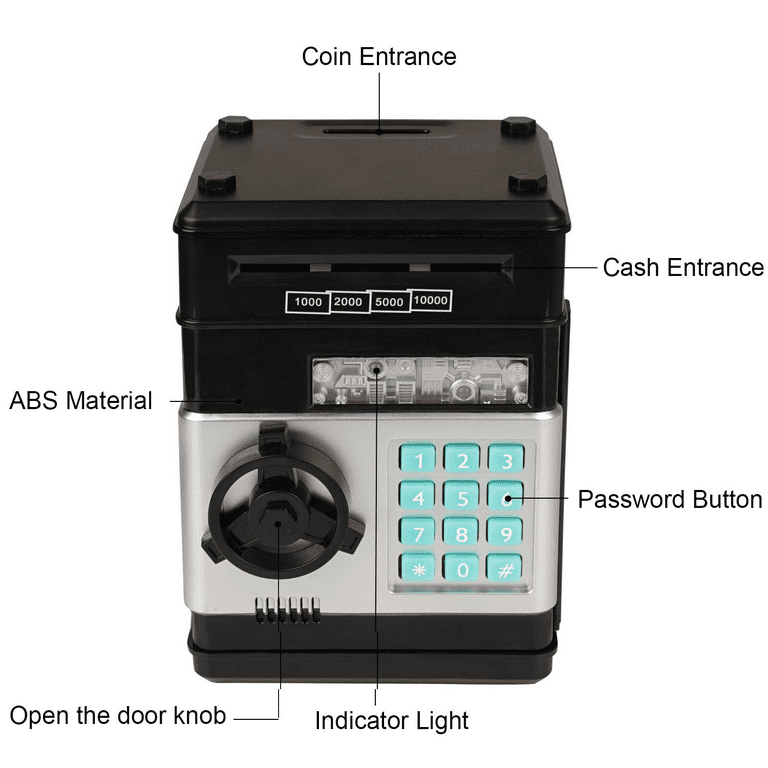The photograph showcases a black coin vault with a prominently featured silver keyboard at its center, surrounded by clear gears visible through a transparent section. These gears are located above the keypad, which is composed of small cyan square buttons arranged like a telephone keypad with white numbers. Each button is numbered 1-9, with the fourth row including a diamond, 0, and the pound symbol. The keypad's "Password Button" label points to the number 6. 

To the left of the keypad is a small black doorknob, labeled "Open the Doorknob," indicating it can be twisted to operate the safe. An indicator light is situated near the clear gears, denoted as being made of ABS material. The vault also features a hopper entrance for coins located at the top center, referred to as the "coin entrance." On the right side of the unit, a label points to a slot identified as the "cash entrance." This slot runs horizontally along the side of the safe. The overall design suggests it is a functional yet lightweight device, possibly intended for a child's use.